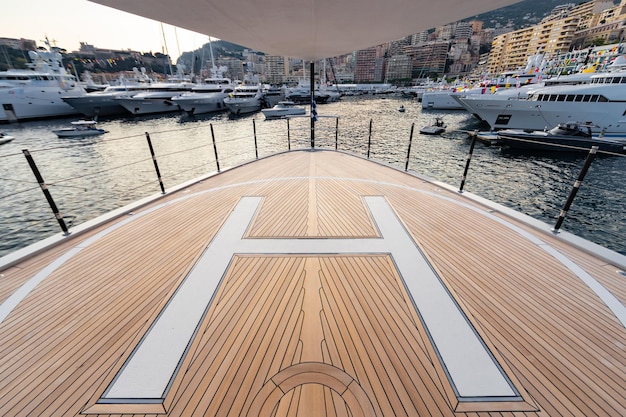In this detailed color photograph, we see the bow of a large yacht, identifiable by its polished inlaid wooden deck and a prominent white "H" outlined in black, encircled by a white ring. The bow's edges are lined with black railings and topped with a white cover. The yacht faces a bustling marina filled with a mix of seven large yachts and smaller boats, predominantly in shades of white, gray, and blue. On the right side of the marina, a distinct black boat stands out amongst the vessels. A rippling bluish-gray water, probably stirred by the activity and wind, fills the foreground. Beyond the marina lies a vibrant cityscape featuring a mix of red, brown, and orange buildings, with some larger structures set into rocky terrain. No people or motorized vehicles are visible, adding to the serene yet lively atmosphere of the scene, captured in broad daylight.